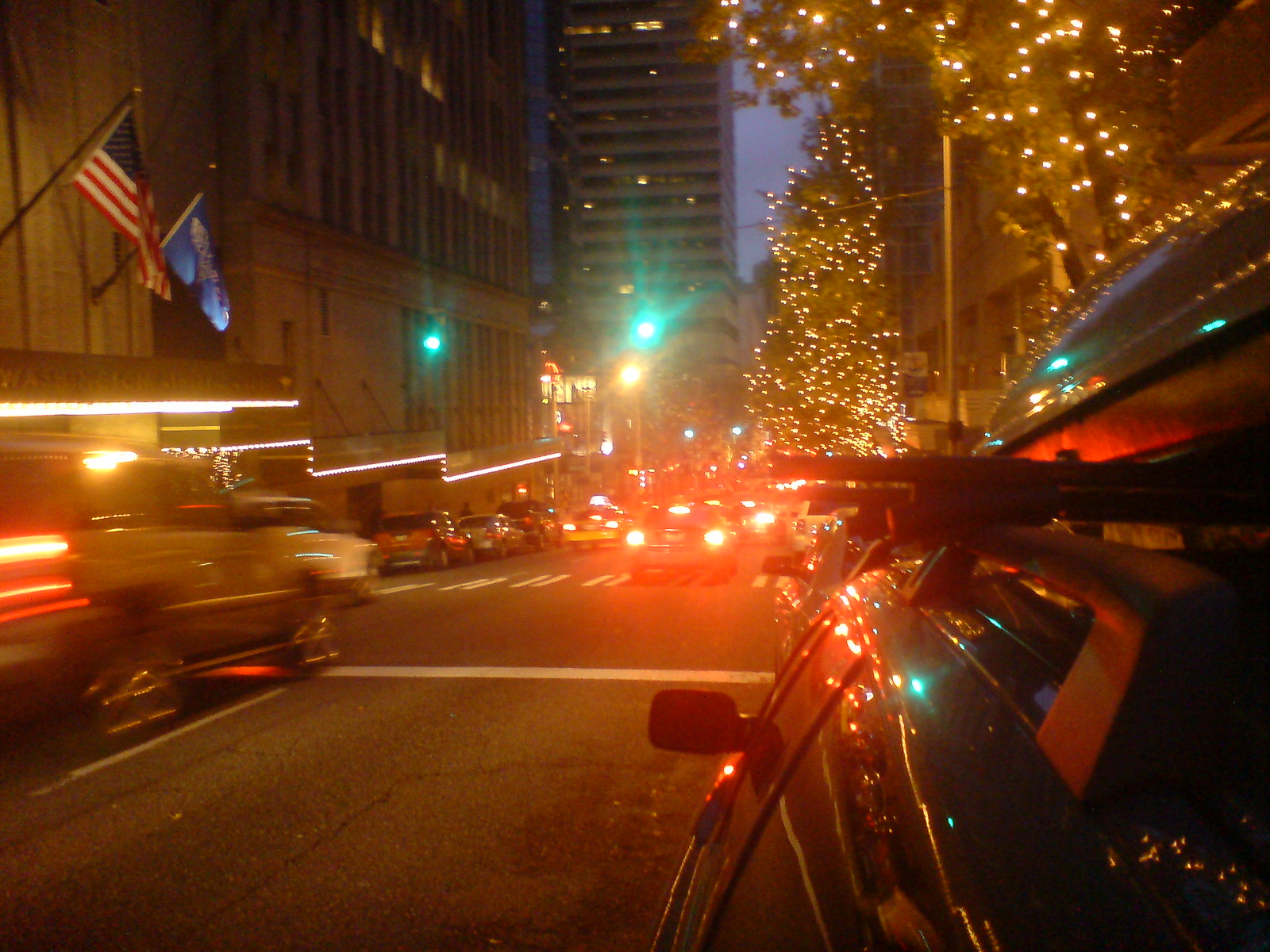A vibrant nighttime photograph capturing the dazzling energy of Times Square in New York City during the holiday season. The image, taken from the perspective of someone extending out from a vehicle window, showcases the bustling atmosphere of this iconic location. The scene is illuminated by an array of vivid colors from the city lights and towering electronic billboards. In the background, a majestic Christmas tree, adorned with twinkling lights, stands proudly amidst the towering skyscrapers of Rockefeller Center. Along the sidewalks, festive trees wrapped in sparkling lights add to the holiday cheer. The photograph also features the bright red glow of brake lights from the dense traffic, enhancing the dynamic feel of the scene. Prominently displayed are an American flag and another national flag, symbolizing the diverse and international spirit of the city.